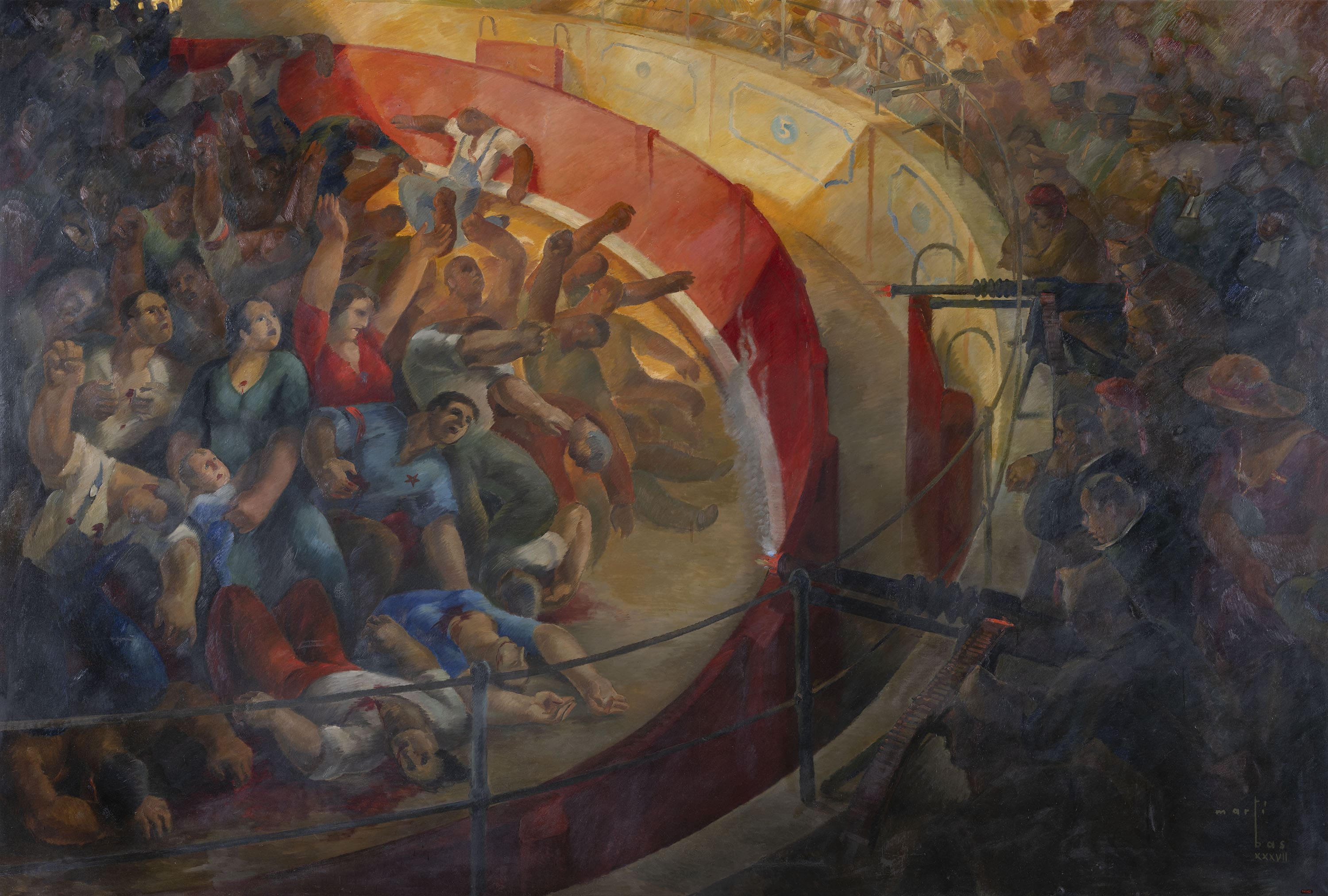The image is a painting with a horizontal orientation, likely inspired by World War II, depicting a disturbing, violent scene set in what appears to be a bullring or coliseum. The crowd of people is confined within a red circular barrier in the center, suggesting they are trapped. Surrounding this red ring is an outer yellowish or gold wall, forming the structure of the coliseum. On the right side of the painting, there's an audience observing the chaos, and in front of them, closer to the red barrier, stand two men with machine guns. The machine gunners are seen actively shooting into the crowd, with visible flames protruding from their weapons. Inside the red ring, the people are portrayed in various states of distress—some are already collapsed on the ground and bleeding, while others are still standing, flailing, or suffering from their injuries. The painting has a cartoony vibe, which adds an eerie, unsettling feel to the violent imagery. The horrifying details, including bullet holes and blood, underscore the grim atmosphere of the scene.